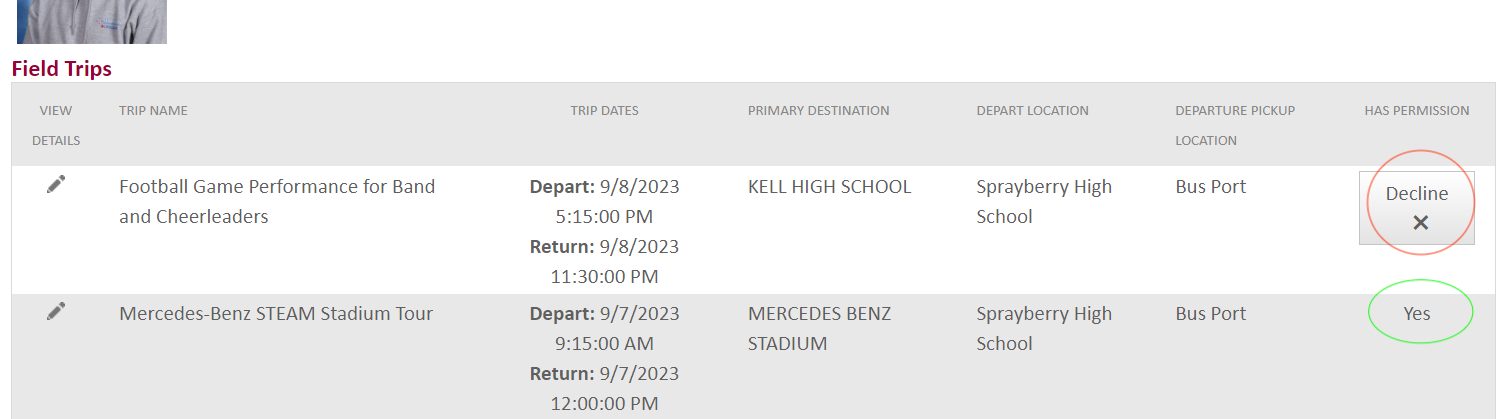**Caption:**

A detailed look at a school field trip receipt is presented in the image. In the upper left corner, there is a square featuring a partial portrait of an individual wearing a gray polo shirt adorned with a blue logo over the left chest. The background of this square is blue. Below the image, in bold red text, the words "Field Trips" are prominently displayed.

The main part of the receipt consists of a printout arranged in a pattern of alternating gray and white bars. The top gray bar acts as the header, listing the columns: *View Details*, *Trip Name*, *Trip Dates*, *Primary Destination*, *Depart Location*, *Departure Pickup Location*, and *Has Permission*.

Under the *View Details* column, a small gray pencil icon is visible. Moving from left to right, the first row details a trip titled "Football Game Performance for Band and Cheerleaders," scheduled to depart on September 8, 2023, at 5:15 PM and return on the same day at 11:30 PM. The primary destination is Kell High School, and the departure locations include Spailbury High School and the busport. The *Has Permission* column for this trip shows a gray box with the word "Decline" and a black "X" underneath, circled in red.

The second row also begins with a pencil icon and provides information about a "Mercedes-Benz Steam Stadium Tour." This trip is set to depart on September 7, 2023, at 9:15 AM and return at 12:00 PM on the same day. The primary destination is Mercedes-Benz Stadium, with the same departure locations as the previous trip. The *Has Permission* column for this trip indicates "Yes," and it is circled in green.